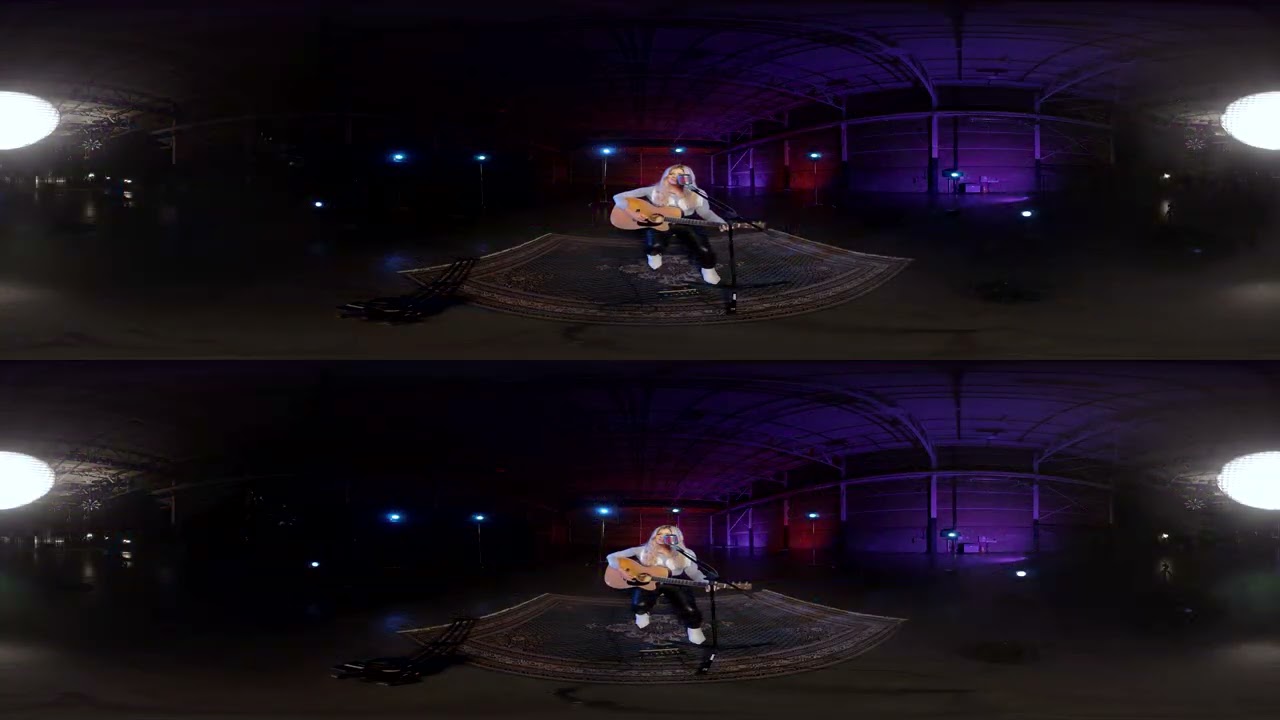In this split-screen image composed of two nearly identical photos stacked one above the other, we see a woman performing with a guitar, seated on a chair, and singing into a microphone on a stand. The setting appears to be a dimly lit warehouse or building with a variety of colored lights, including hues of violet, blue, and red, casting a moody ambiance. Nearby, there's a keyboard visible to the side, indicative of a musical performance. The woman, the focal point, is positioned on a rug with a brownish-gray hue. The overall scene suggests an intimate setting, possibly for a small audience, with the performance captured in two slightly different moments. The background retains a rich mixture of colors, enhancing the visual depth of the location.